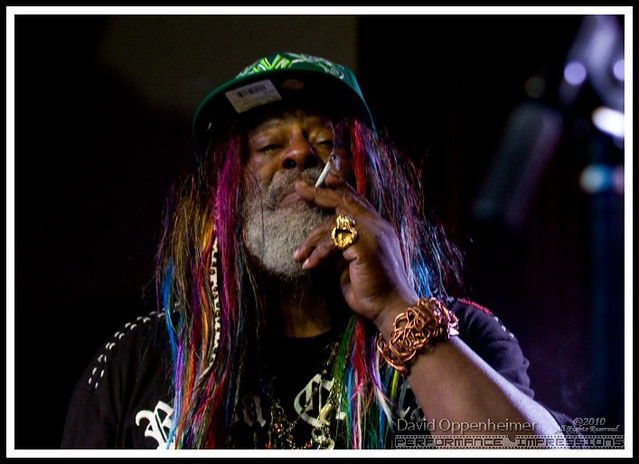This color photograph captures a man with a long, thick, multicolored dreadlocked hair adorned with shades of pink, blue, red, orange, and green. He sports a green baseball cap and boasts a bushy, white beard and mustache. He is gazing directly at the camera with a lit cigarette or joint in his left hand, which is raised to his mouth, emitting visible smoke. On his left hand, he wears prominent rings on both his pinky and the adjacent finger, along with a noticeable copper bracelet made of twisted wire on his wrist. The man is dressed in a black T-shirt featuring white lettering, partially obscured by his vibrant hair. In the lower right-hand corner of the image, white text reads "David Oppenheimer, 2016" or "2010." The background primarily features a black backdrop with an out-of-focus microphone positioned in the upper right-hand corner.